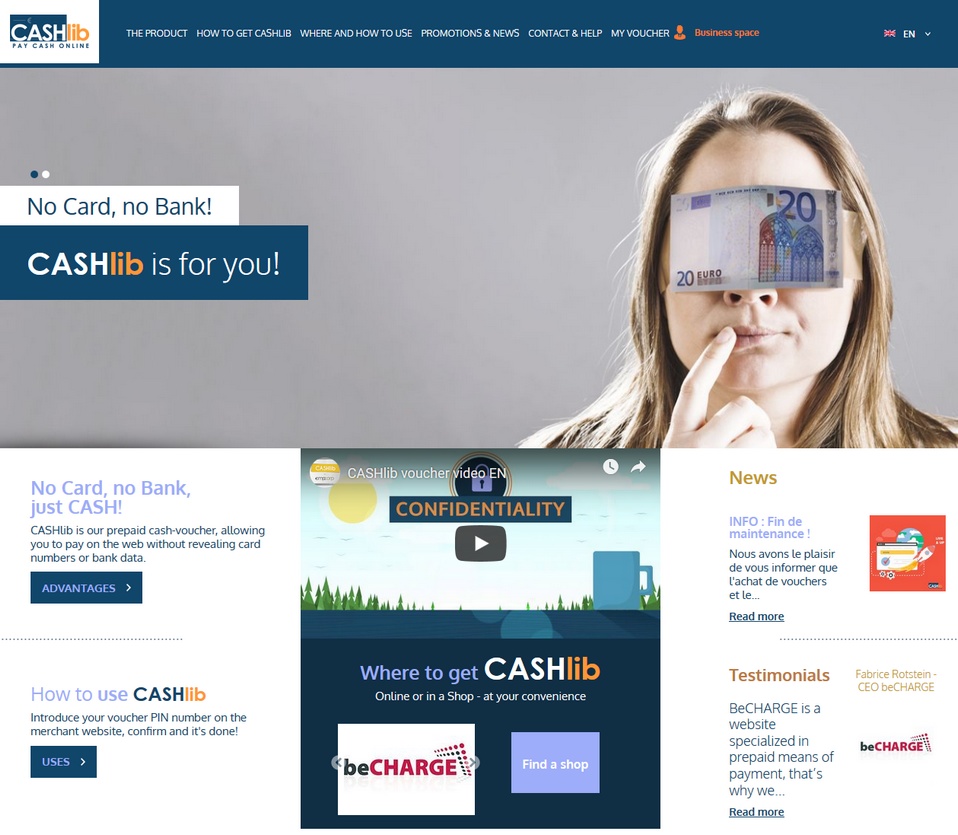**Detailed Caption:**

The screen capture displays a webpage for "Cashlib - Pay Cash Online." In the top left corner, there's a logo for the service. To the right, a menu bar includes several options: "The Product," "How to Get Cashlib," "Where and How to Use," "Promotions and Uses," and "Contact and Help." An orange-highlighted section labeled "My Voucher" is also visible. On the far right, there's a language selection dropdown currently set to English (EN) with a British flag icon.

Beneath the menu, a large image spans the page with a grey background. On the right side of this image, there's a woman with a pensive expression, holding a finger to her lips, and a €20 note is covering her eyes. To the left of the woman, bold text on a white and blue backdrop declares, "No Card, No Bank! Cashlib is for YOU!"

Further down, the layout is divided into multiple sections. On the left, two white-background boxes provide information, while two more are on the right. Centrally, a video box is prominently displayed. Below, text on a dark blue background reads, "No Card, No Bank, Just Cash," followed by details about Cashlib and a clickable button labeled "Advantages." Dotted lines separate different informational blocks.

One section titled "How to Use Cashlib" includes instructions and another button for more detailed uses. Another highlighted box on the right offers "News Info" with text in French and a "Read More" option, accompanied by a red image featuring a globe and stylized computer screen.

Below these sections, testimonials are displayed, including one from "BeCharge," a website specializing in prepaid payment methods with a brief description and a "Read More" link. An image next to this displays the "BeCharge" logo with additional foreign text.

The central video box includes the title "Cashlib Voucher Video EN" with an image of a padlock at the top and a banner reading "Confidentiality." A play button is overlaid on a scene depicting a sun in a blue sky, pine trees, and a blue mug.

Finally, text on a dark blue background at the bottom emphasizes, "Where to get Cashlib: Online or in a Shop at Your Convenience," with a white square featuring "BeCharge" and a purple square prompting users to "Find a Shop."